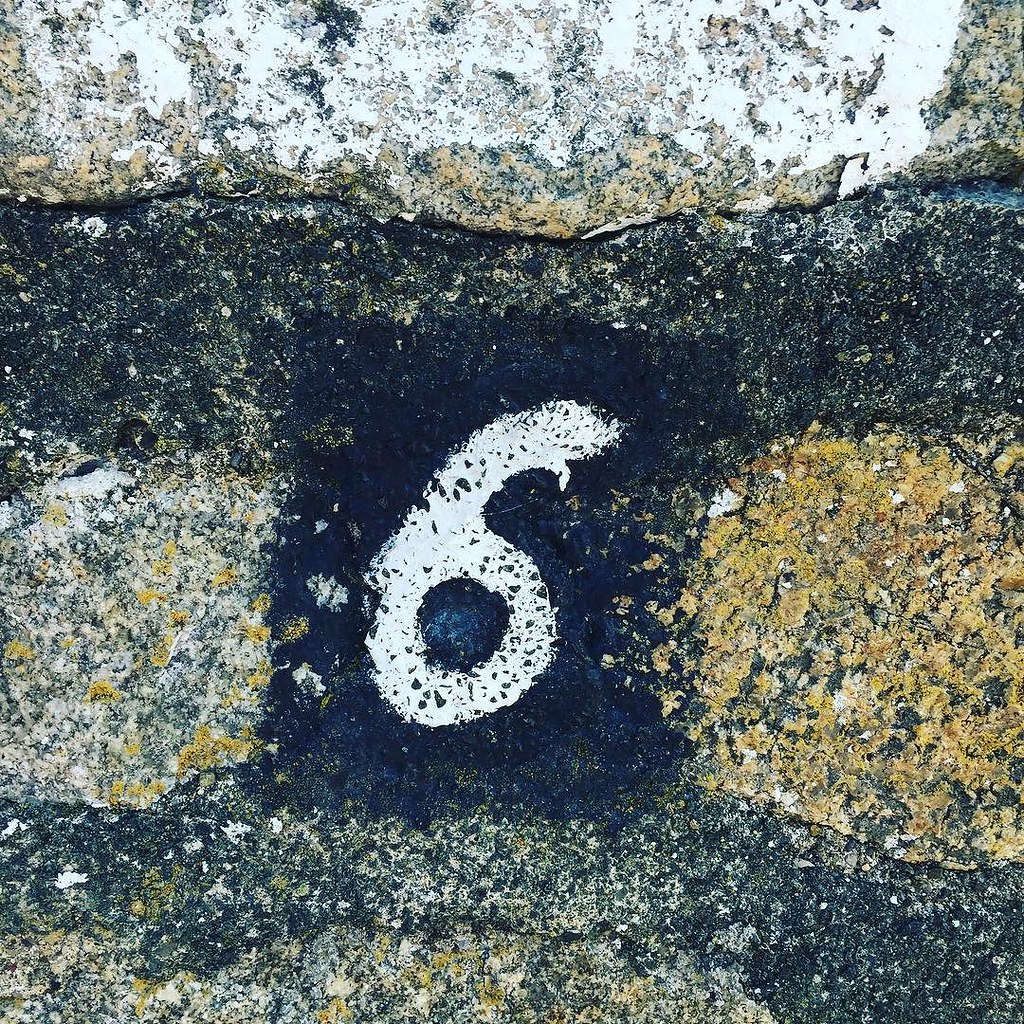This photograph captures an up-close view of a number six painted in white on a black rectangular background. The background and the six are set against a worn pavement, likely part of a roadway. The pavement shows signs of wear and aging, revealing a mixture of faded colors and materials. Surrounding the black rectangle, remnants of what used to be a yellow line, now largely worn off and mixed with black tar patches, are visible. The area to the left of the six shows a transition from the old yellow line to more recent white paint, while the right side retains some yellow but is largely marred by the underlying black tar. Beneath the six, additional faded yellow suggests the former existence of a double line. At the top of the image, a chipped and faded white line possibly indicates the edge of a curb. The road's surface exhibits a grainy texture with shades of charcoal gray, light gray, and tan, hinting at the use of gravel or cement material. The setting appears to be outdoors, on a cement or gravel roadway, with the number six prominently centered within the composition.